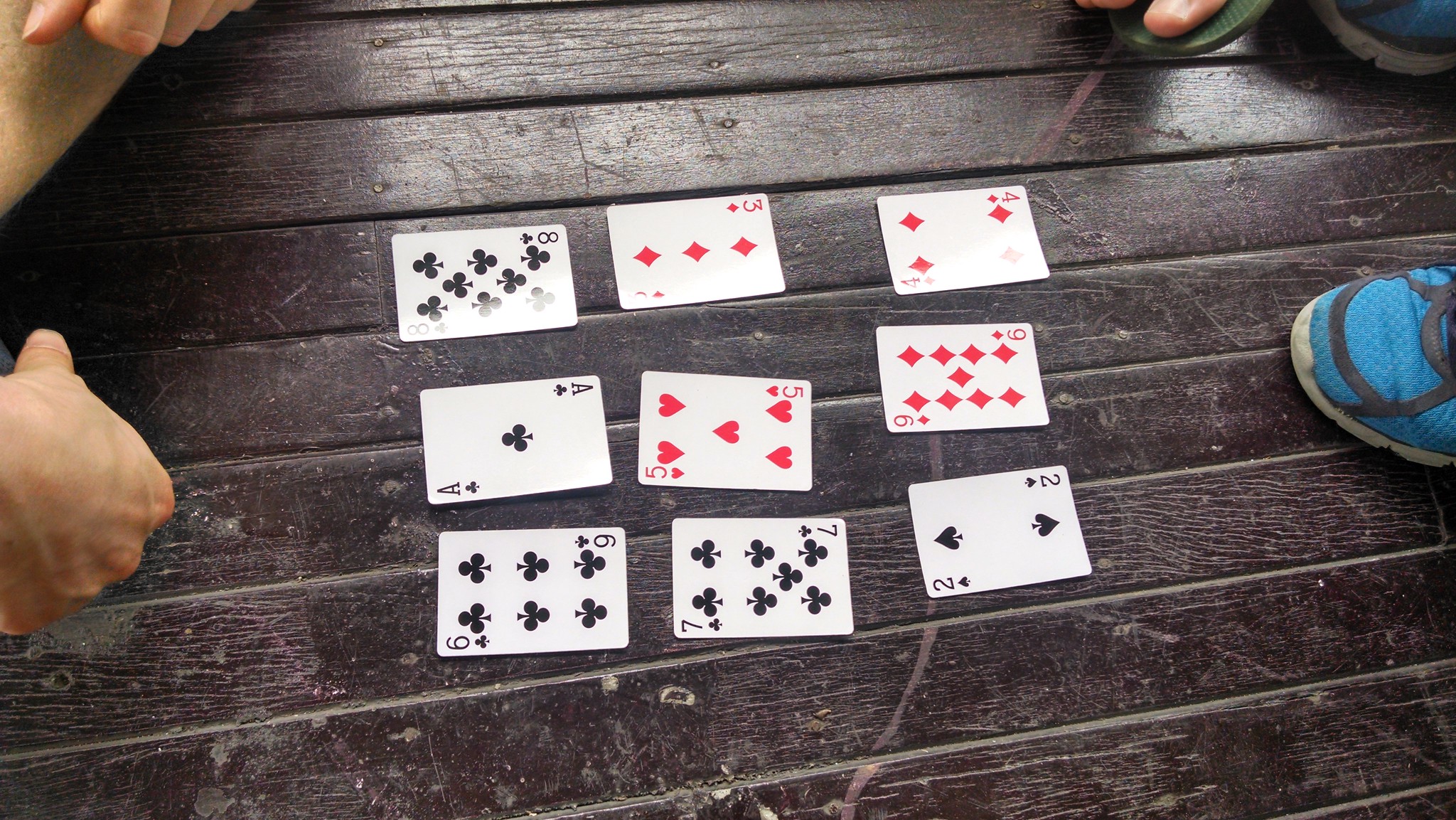In this photograph, nine playing cards are meticulously arranged in a 3x3 grid on a rough, somewhat dirty wooden floor. The floor's texture and grime add a raw, rustic quality to the image. Surrounding the cards are several individuals, their presence only hinted at by glimpses of their hands and feet. In the lower left corner, there is a partial view of a hand with the thumb and knuckle visible, while the fingers remain out of the frame. On the top left, another person's hands rest on their knees, positioned in a way that suggests they are sitting cross-legged, with both hands slightly bunched into fists.

On the opposite side of the card layout, you can spot the blue sneakers of another individual and a portion of their hand. The cards, laid out in an east-west direction, from left to right in each row, are as follows: 

- Top row: Eight of Clubs, Three of Diamonds, Four of Diamonds.
- Middle row: Ace of Clubs, Five of Hearts, Nine of Diamonds.
- Bottom row: Six of Clubs, Seven of Clubs, Two of Clubs.

The exact game these individuals are playing remains a mystery, but their focused arrangement suggests an engaging activity that demands their attention to the cards spread before them.